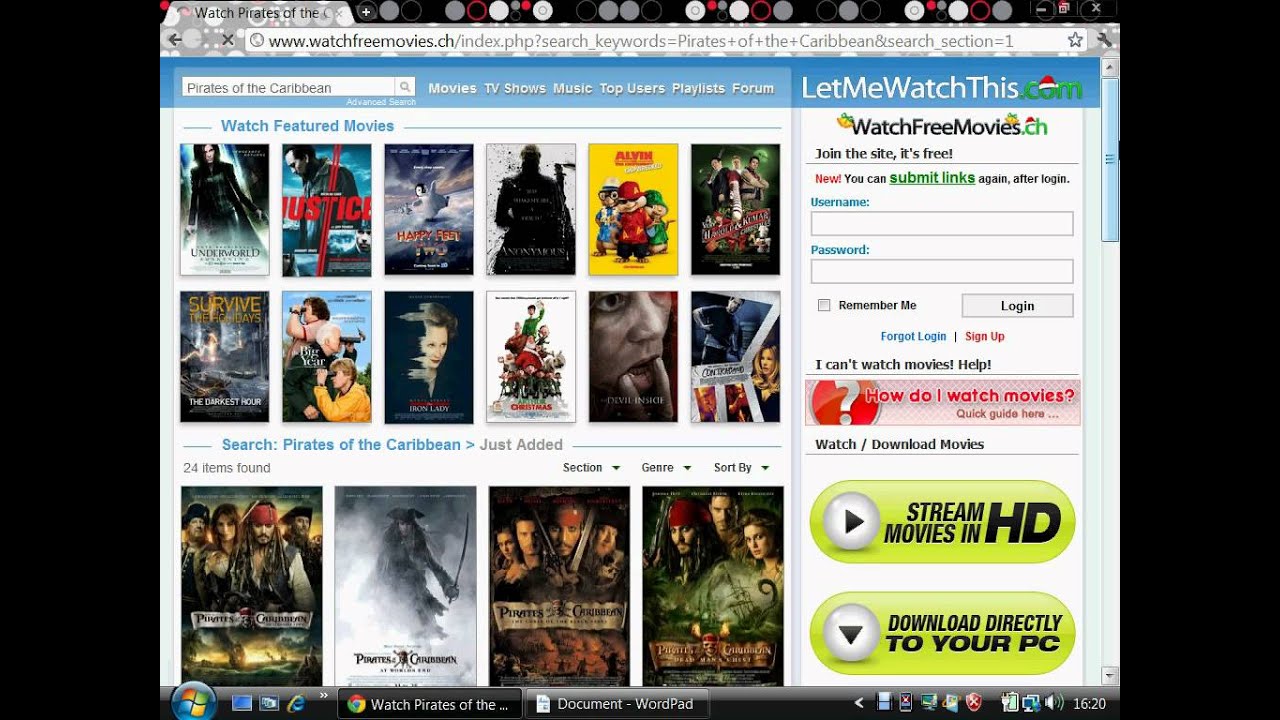A screenshot of a desktop computer displaying an open web browser on LetMeWatchThis.com. The page features a search for "Pirates of the Caribbean," resulting in a list of 24 items. Prominently displayed are four different movie posters from the "Pirates of the Caribbean" series, showcasing various movie artworks. The website, set against a primarily white background, features a blue search bar at the top and entry fields for username and password. Additional advertisements are visible along the sides.

The desktop's taskbar reveals several active applications, including a Chrome browser (identified by its colorful circular logo), Internet Explorer, and WordPad. The bottom right corner of the taskbar presents system indicators like antivirus software, a Windows Update icon, battery percentage, volume controls, and the current time. The iconic multi-colored Windows logo (orange, green, blue, and yellow) is also visible.